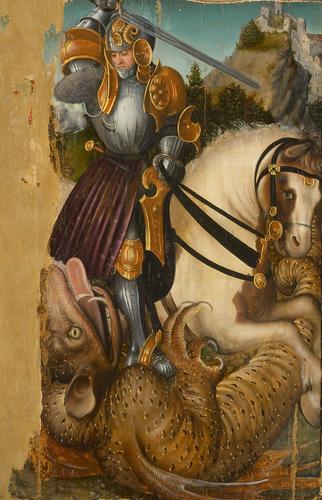The painting vividly depicts a knight on a white horse, gripping black reins that extend from the horse's mouth to his armored hands. The knight's armor is predominantly silver metal, embellished with gold plating on his shoulders, elbows, and knees, and a red waist cloth or cape adds a striking contrast. With a stoic expression, he raises his sword high against the sky, poised to deliver the final blow to a dragon-like beast beneath him. The dragon, covered in tan and brown scales, has small wings, long ears, horns, and a tail that curls under the horse. Its mouth is open in a cry, revealing both upper and lower fangs, and its tongue protrudes slightly. The beast's clawed hands are positioned in a peculiar A-OK gesture. In the background, a castle perched on a distant hill completes the medieval scene, which is richly painted in vivid warm colors like red and green. The dramatic tension centers on the knight, who uses his left foot to hold the dragon down as he prepares to strike.